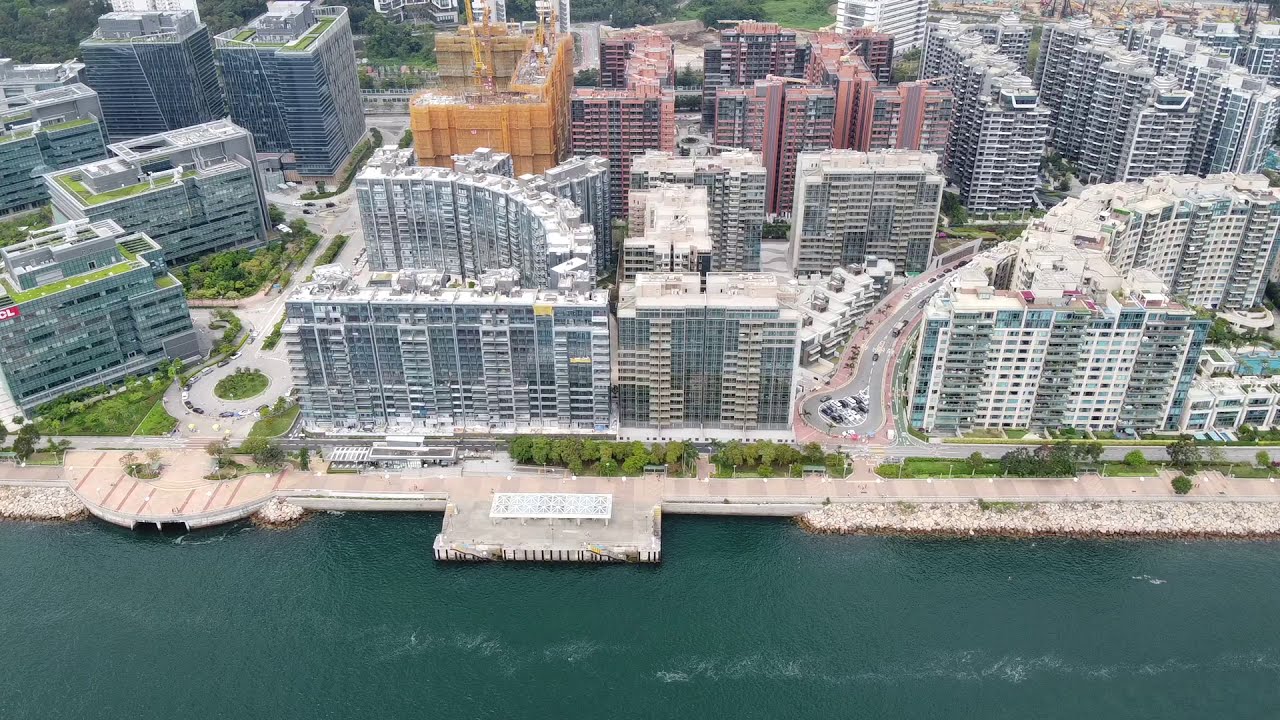This aerial view of a large metropolitan city reveals a dense cluster of high-rise buildings ranging from about 15 to 40 stories, comprising of apartments, hotels, and office buildings. The buildings, in a palette of orange, red, and blue with predominantly white roofs, form tightly knit complexes interspersed with green spaces. Surrounding these structures are grass fields, trees, and intertwined roads. The cityscape extends towards a waterfront featuring a green-blue river, where a boat stirs ripples on its surface. On this clear, sunny day, the riverbank is lined with lush bushes and trees, enhancing the natural beauty amidst the urban environment.